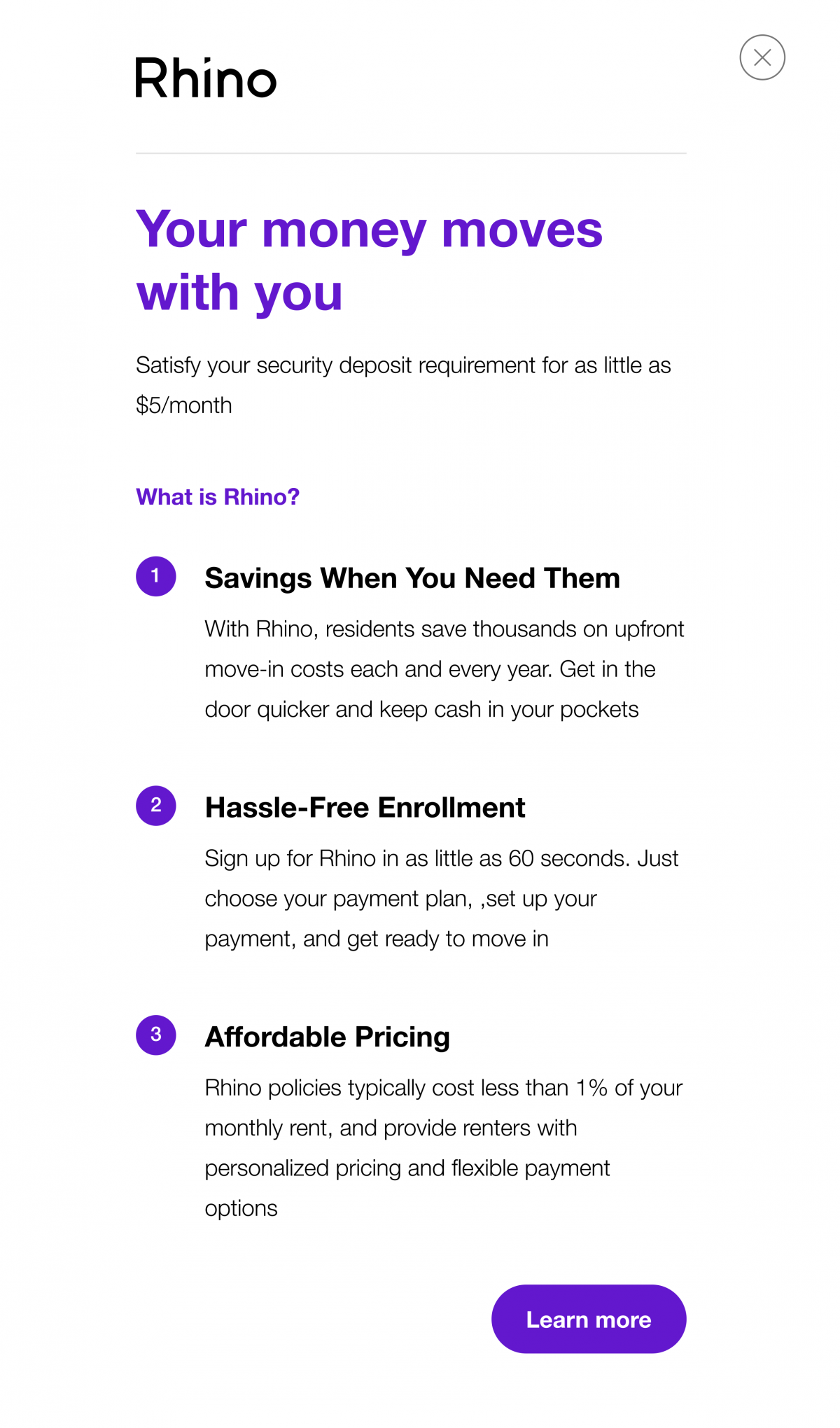Here we have a screenshot from a mobile phone screen featuring a predominantly white background. Absent are the usual status bar indicators at the top, creating a clean and minimal look. At the very top of the image, above a grey line, the word "RINO" appears in bold black font, aligned to the left. To the right of "RINO," there's a grey circle with an "X" inside it, indicating an option to close or exit out of the current screen.

Beneath this header, in bold purple font, the text "Your Money Moves With You" stands out prominently. Below this, in a very small and non-bolded black font, the text reads, "Satisfy Your Security Deposit Requirement for as little as $5 a month." In a slightly larger, purple font, the question "What is RINO?" appears, potentially bolded, inviting further exploration.

The main body of the content is structured into three sections, each introduced by a logo and a bold numerical heading:

1. **Savings When You Need Them**: This section is introduced with bold, dark black font, explaining how "With RINO, residents save thousands on move-in costs each year. Get in the door quicker and keep cash in your pockets."

2. **Hassle-Free Environment**: This section describes how one can "Sign up for RINO in as little as 60 seconds. Just choose your payment plan, set up your payment, and get ready to move in."

3. **Affordable Pricing**: This final section, also in black font, notes, "RINO policies typically cost less than 1% of your monthly rent and provide renters with personalized pricing and flexible payment options."

At the bottom of the screen, there's a prominent purple button labeled "Learn More" in white font, inviting users to obtain additional information.